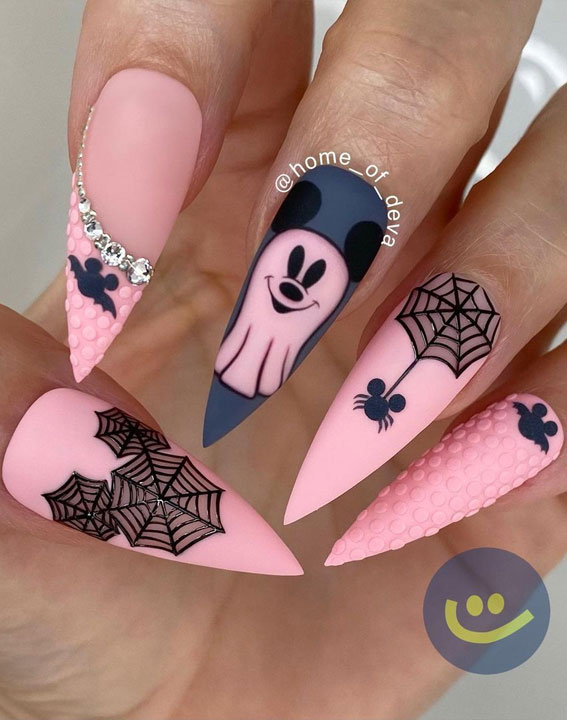This close-up photograph showcases a black woman's hand, emphasizing her elaborately designed, pressed-on acrylic nails. The nails are long, sharp-pointed, and predominantly feature a pink background, except for the middle finger, which has a dark gray base. Each nail flaunts a unique Halloween-themed design. The woman's thumbnail is adorned with intricate black spider webs. The index finger sports a swish of rhinestones traversing from top to middle, overlaying textured pink polka dots and a black bat. The standout middle finger displays a large pink sheet ghost with Mickey Mouse ears. The ring finger features a black spider web with a dangling spider, also incorporating a Mickey Mouse theme. Lastly, the pinky finger has a bat motif perched on its pink base. Her fingers are curled over her palm, presenting all nails clearly in the tightly zoomed-in image, revealing the varied and detailed artistry of her manicure.